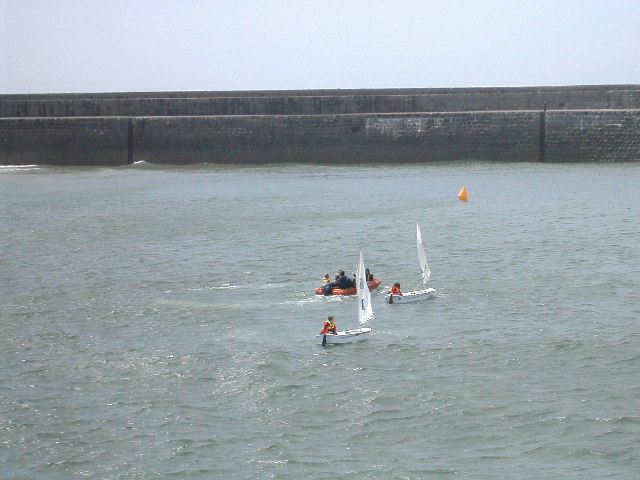The photograph captures a daytime scene of a calm, bluish-gray body of water, likely a bay or ocean. In the foreground, there are two small white sailboats, each with a person wearing a life jacket, and white sails. Nearby, an orange inflatable raft floats with several people aboard, likely five or six, some of whom are also wearing life jackets. The water shows a mix of calm areas and some gentle waves closer to a tall, gray stone retaining wall that spans the background of the image; this wall appears to function like a seawall or break-wall. Off in the distance, a yellow flag is visible on the water. Additionally, an orange buoy and a red motorized boat with about seven to eight people can be seen, emphasizing the scene's dynamic aquatic activities. The stone barrier, possibly a bridge or seawall, has a two-tiered structure, creating a sense of depth and distance, with a glimpse of one small figure standing on it.